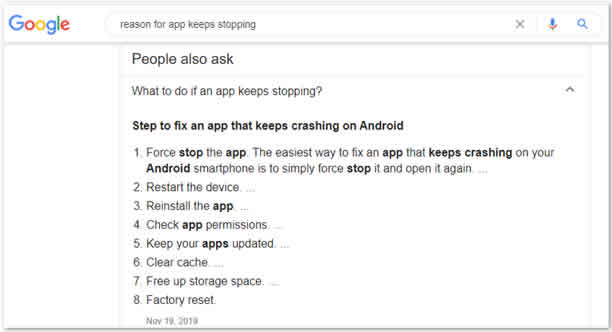The image appears to be a screenshot taken from a computer. In the upper left corner, the recognizable Google logo is displayed, featuring the word "Google" in its signature blue, red, yellow, and green colors. Adjacent to the logo is a search bar containing the query: "reason for app keeps stopping". 

The primary section of the screenshot has a white background with a prominent rectangle situated on the right side. At the top-left corner of this rectangle, the heading "People also ask" is written in black font. Beneath this heading, there is a question inquiring, "What to do if an app keeps stopping?" 

Following this, there is a highlighted section titled "Steps to fix an app that keeps crashing on Android." This section provides an organized list of eight steps to resolve app crashing issues. The steps are as follows:

1. **Force stop the app**: The explanation provided suggests that the simplest way to troubleshoot a crashing app on an Android device is to force stop the app and then reopen it. The words "stop" and "app keeps crashing on Android" are emphasized in dark black text.
2. **Restart the device**.
3. **Reinstall the app**: The word "app" here is highlighted in black text.
4. **Check app permissions**: Similar to step 3, the word "app" is in dark black.
5. **Keep your apps updated**: The word "apps" is emphasized in dark black text.
6. **Clear cache**.
7. **Free up storage space**.
8. **Factory reset**.

The detailed steps conclude with a date at the bottom, indicating "November 19th, 2019."